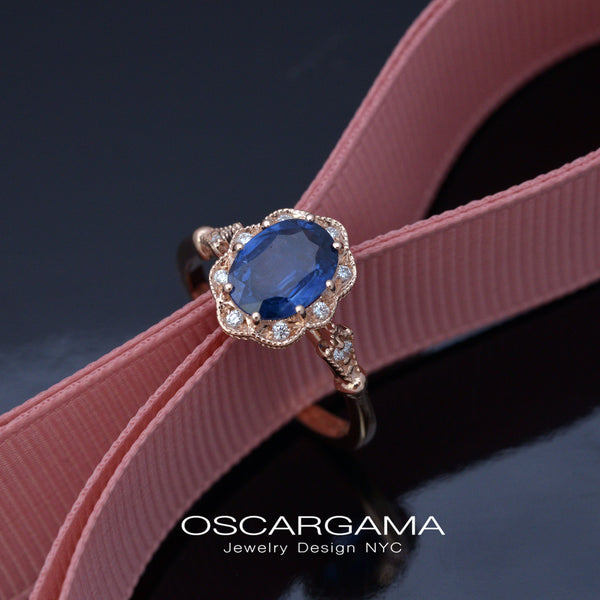The advertisement features a luxurious, antique-inspired ring by Oscar Gamma Jewelry Design NYC. The focal point is a captivating deep blue sapphire, elegantly set with eight mounts and encircled by dazzling diamonds on a circular gold mount. The ring, with its exquisite craftsmanship, is threaded through a striking pink, almost dark peach-colored strap, adding a unique touch to the display. Beneath the ring, the designer's name, "Oscar Gamma," is prominently displayed in white letters, followed by the smaller text "Jewelry Design NYC." The entire composition is set against a dark blue, nearly black mirrored background, highlighting the opulence and sophistication of the ring, which could easily be seen as a stunning engagement piece.